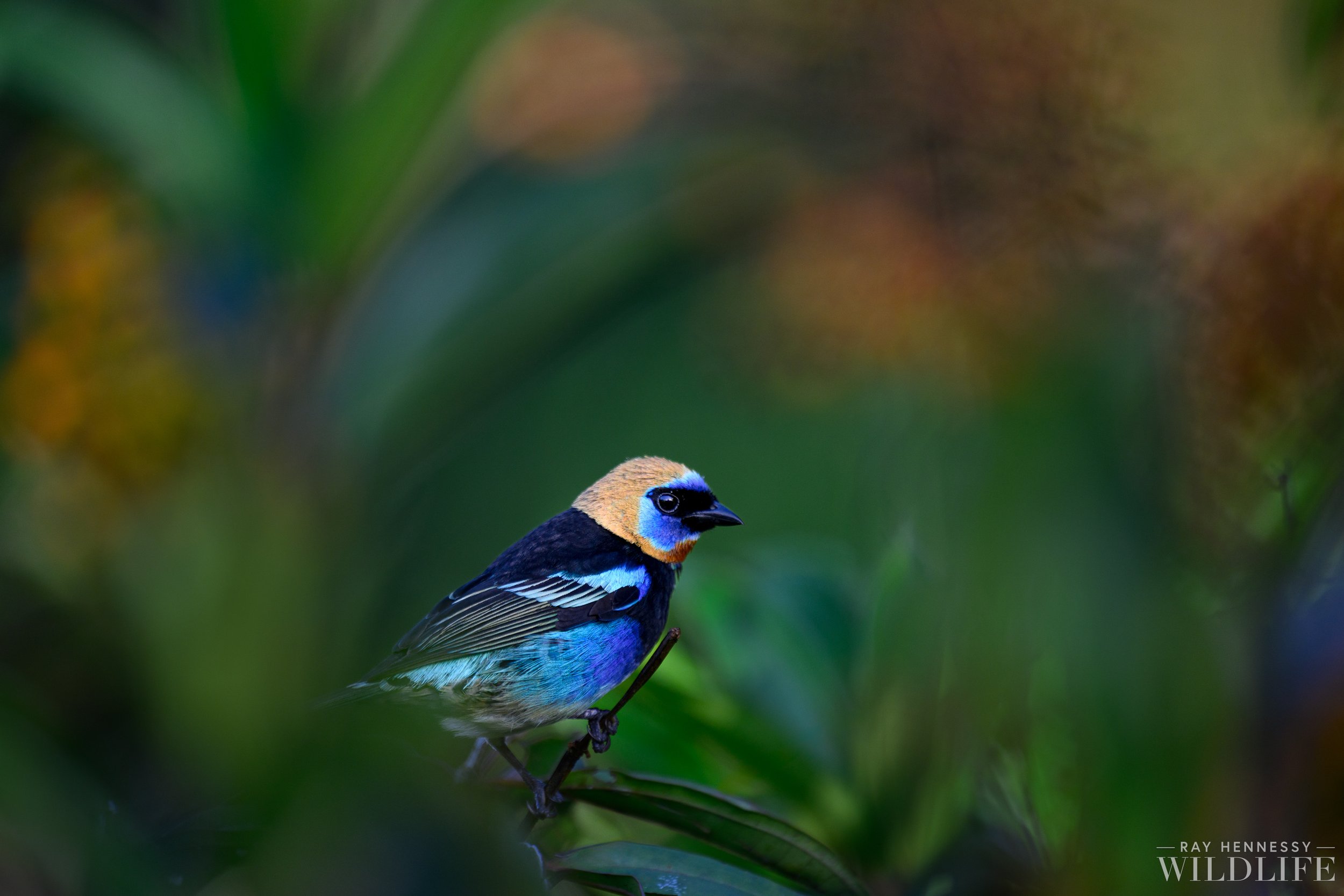This close-up photograph showcases a striking golden-hooded tanager, a medium-sized passerine bird found from southern Mexico to western Ecuador. Perched on a small, dark green branch flanked by similarly colored leaves, the tanager's vibrant plumage is a feast for the eyes. Its head is a pastel orange, transitioning to a stunning cyan and dark blue face, with sharp black outlines around the eyes and a small, dark blue beak. The bird's wings display an intricate pattern of shades of blue, featuring stripes of cyan, dark blue, and white, with accents of green towards the tail feathers. The back and body are primarily dark blue, blending into lighter blue and cyan towards the lower body and feet. The background is an artistic blur of natural colors—spots of dark and light green, yellow, olive, beige, dark brown, and light brown—giving the scene a dreamy, almost painted quality. In the lower right-hand corner, the white text reads, "Ray Hennessey Wildlife," with "Hennessey" spelled H-E-N-N-E-S-S-Y, marking the photographer's credit. The photograph, taken in daylight, captures the stark beauty of the tanager in its natural habitat.